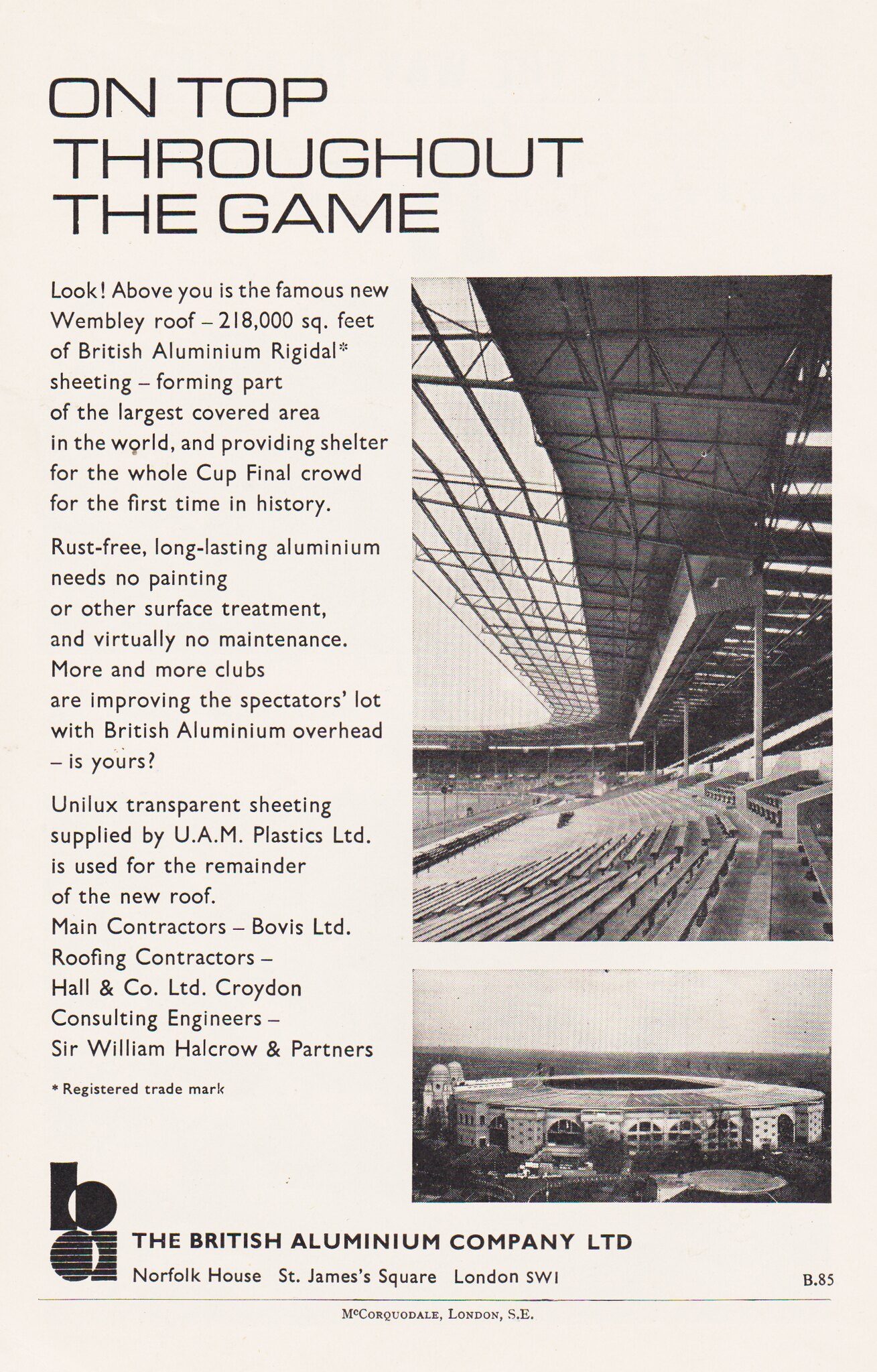The image is a full-page magazine advertisement with a white background featuring two black-and-white photographs. The headline, in thin sans-serif font, reads "On Top Throughout the Game." Along the left side of the page, there is a column of black text detailing the attributes of the new Wembley Stadium roof, which is made of 218,000 square feet of British aluminum Rigadale sheeting. This remarkable structure forms the largest covered area in the world, providing shelter for the entire cup final crowd for the first time in history. The advertisement emphasizes the rust-free, durable nature of the aluminum, which requires no painting or significant maintenance. Additionally, Unilux transparent sheeting, supplied by UAM Plastics Ltd., is used for the rest of the roof.

The right side of the advertisement displays two black-and-white photographs. The top image is a vertical rectangle showing the upper-level seating area of the stadium, with rows of seats and the roof overhead. Below it, a horizontal rectangular photograph gives an exterior view of the stadium from a distance. At the bottom of the page, there's a logo in black and white consisting of circles and vertical rectangles. To the left of the logo, in bold print, it reads "The British Aluminum Company Limited," with an address, "Norfolk House, St. James Square, London SW," in smaller, hard-to-read text. In the far right corner of the page, there is an indistinguishable page number.